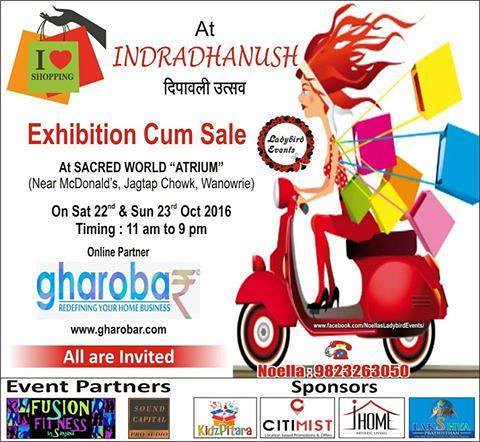The image is a promotional poster for the Indrahanuj "I Heart Shopping Exhibition Come Sale" at the Sacred World Art Atrium near McDonald's Jagtop Chowk. The event is scheduled for Saturday, October 22nd, and Sunday, October 23rd, 2016, from 11 AM to 9 PM. The poster features a digitally produced graphic of a woman riding a scooter on the right side, laden with several shopping bags. The background of the poster is vibrant with colors like white, orange, green, black, red, pink, hot pink, yellow, blue, and purple. The event is hosted by Lady Bird Events, with online partner Garoba Redefining Your Home Business. Other sponsors and partners include Fusion Fitness, Sound Capital, City Mist, iHome, and Kids Pitara. The detailed and colorful design emphasizes the excitement and variety expected at the exhibition.